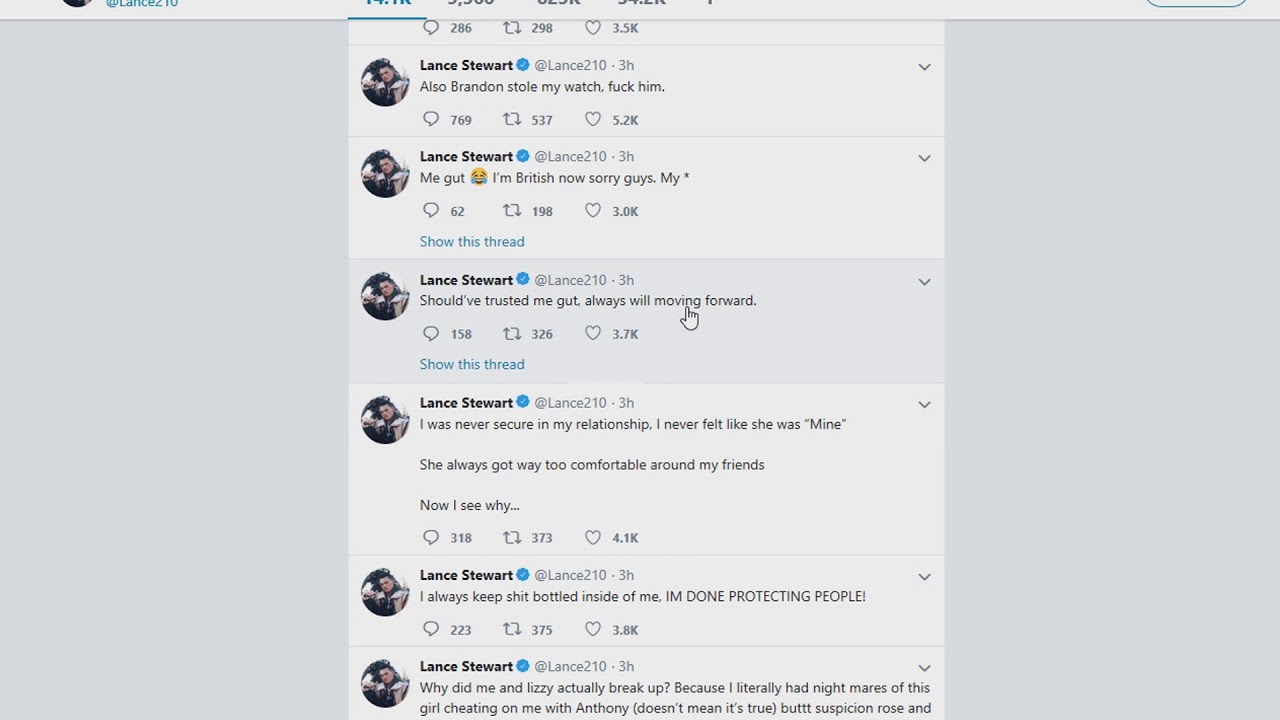The image appears to depict a screenshot of what seems to be a Twitter feed, speculated to be proportionally wider than it is tall, likely around 50% wider. The image is flanked by darkened areas on the left and right, each occupying roughly 30% of the total width. At the very top, there's a light gray horizontal menu bar, hinting at it being part of a website interface, although only the lower parts of four menu options are visible.

Moving towards the center of the image, the remaining visible area showcases a feed set against a light gray background. This feed consists of six posts authored by Lance Stewart, who is verified on Twitter as indicated by a blue checkmark next to his name. His Twitter handle, @Lance210, is visibly consistent across all posts. 

The individual posts are listed chronologically as follows:
1. Three hours ago, Lance tweeted, "Also Brandon stole my watch, fuck him."
2. Lance tweeted, "Me, gut," followed by a laughing face emoji, and then, "I’m British, now sorry guys, my *star*."
3. Another tweet reads, "Should have trusted me, gut, always will moving forward."
4. Lance tweeted, "I was never secure in my relationship. I never felt she was 'mine'."
5. Finally, he comments, "She always got way too comfortable around my friends."

Each tweet is clearly displayed, revealing a mix of personal reflections and casual updates, providing a candid glimpse into Lance Stewart's thoughts and experiences.